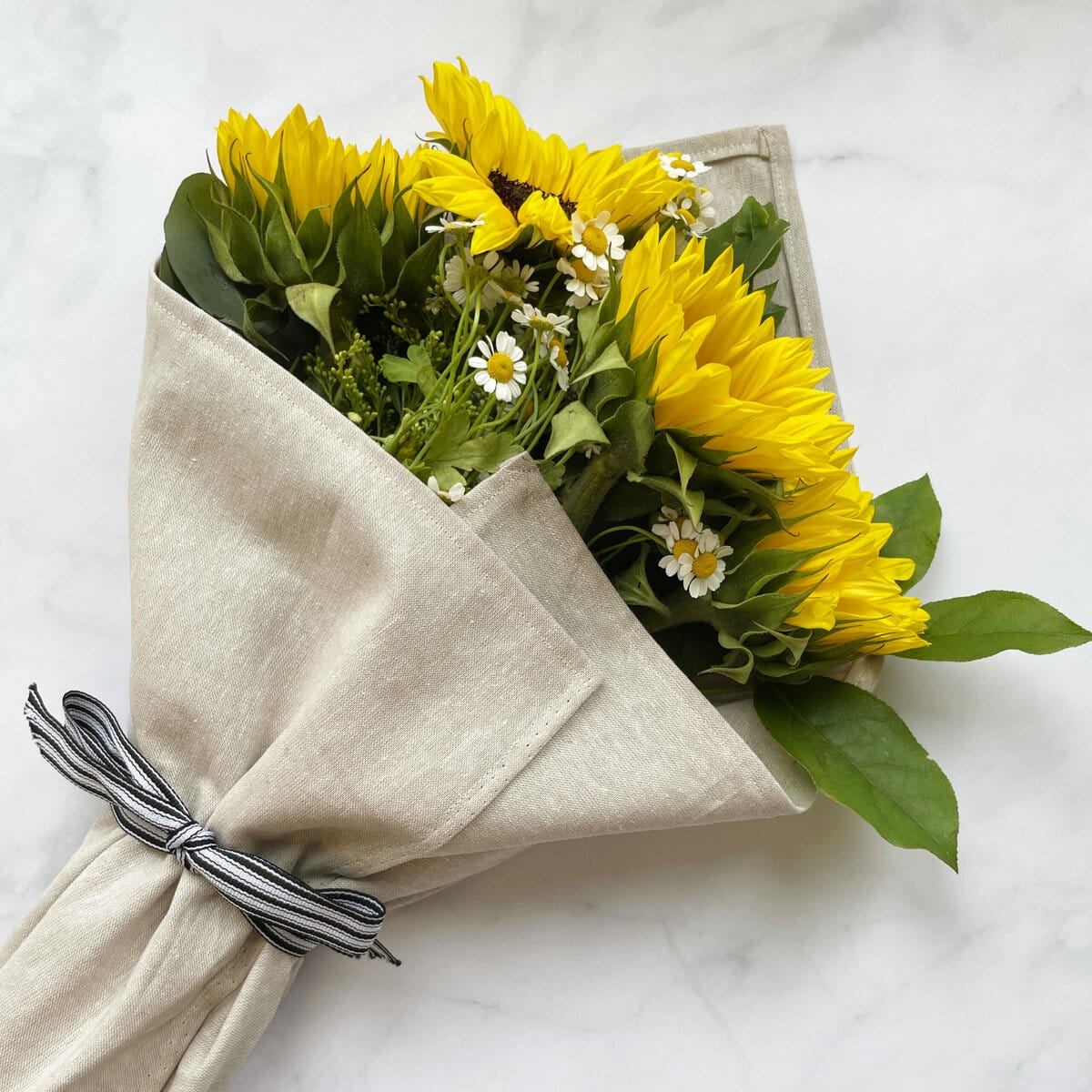This image captures a beautifully arranged bouquet of flowers laid out on a marbled countertop with white and silver veins, viewed from above. The bouquet, which showcases vibrant yellow sunflowers and delicate white daisies with yellow centers, is uniquely wrapped in a cloth, deviating from the typical tissue paper or plastic wrapping. The cloth is elegantly secured with a black and white thinly striped ribbon tied in a bow at the front, about halfway up the bouquet. The arrangement also includes ample greenery, with leaves peeking out from both the right and left sides, adding a touch of freshness to the overall appearance. The setup and presentation suggest it could be part of a how-to guide or a display of a finished floral product, emphasizing its creative and artisanal wrapping.